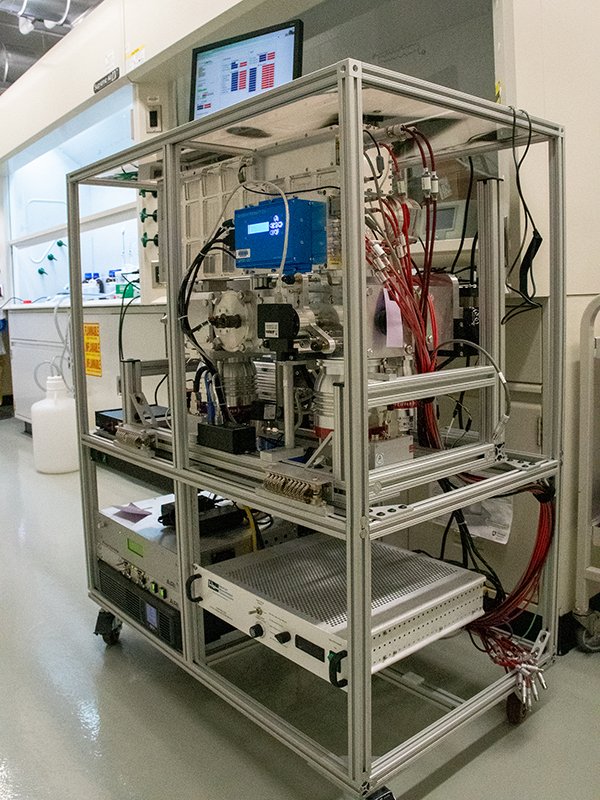The image depicts a tall, metal cart on wheels, likely around six feet in height, situated in what appears to be a hospital hallway or laboratory. The primary piece of equipment on the cart is identified as an aerial mass spectrometer. At the very top of this cart is a computer monitor displaying indistinguishable writing and bar graphs in blue and red. Below the monitor is a substantial blue box and an elaborate array of red and black wires extending from the apparatus. 

The middle section of the cart contains various scientific instruments, including a gray box with dials and a green LCD panel. Another gray box with a different LCD panel is positioned next to it. The bottom section houses more black and silver components with additional control buttons, likened to stereo receiver equipment with numerous dials. The entire setup is interconnected by a complex network of wires.

The cart is positioned on a tile floor, with a large window visible behind it. Adjacent to the cart, on the left, is a brightly lit laboratory bench that may be a sterile hood, containing flasks and tubing, some of which feed into a collection jug on the ground. There is a yellow and red caution symbol on the base of the bench. The entire scene suggests a highly specialized and technical medical or scientific environment.